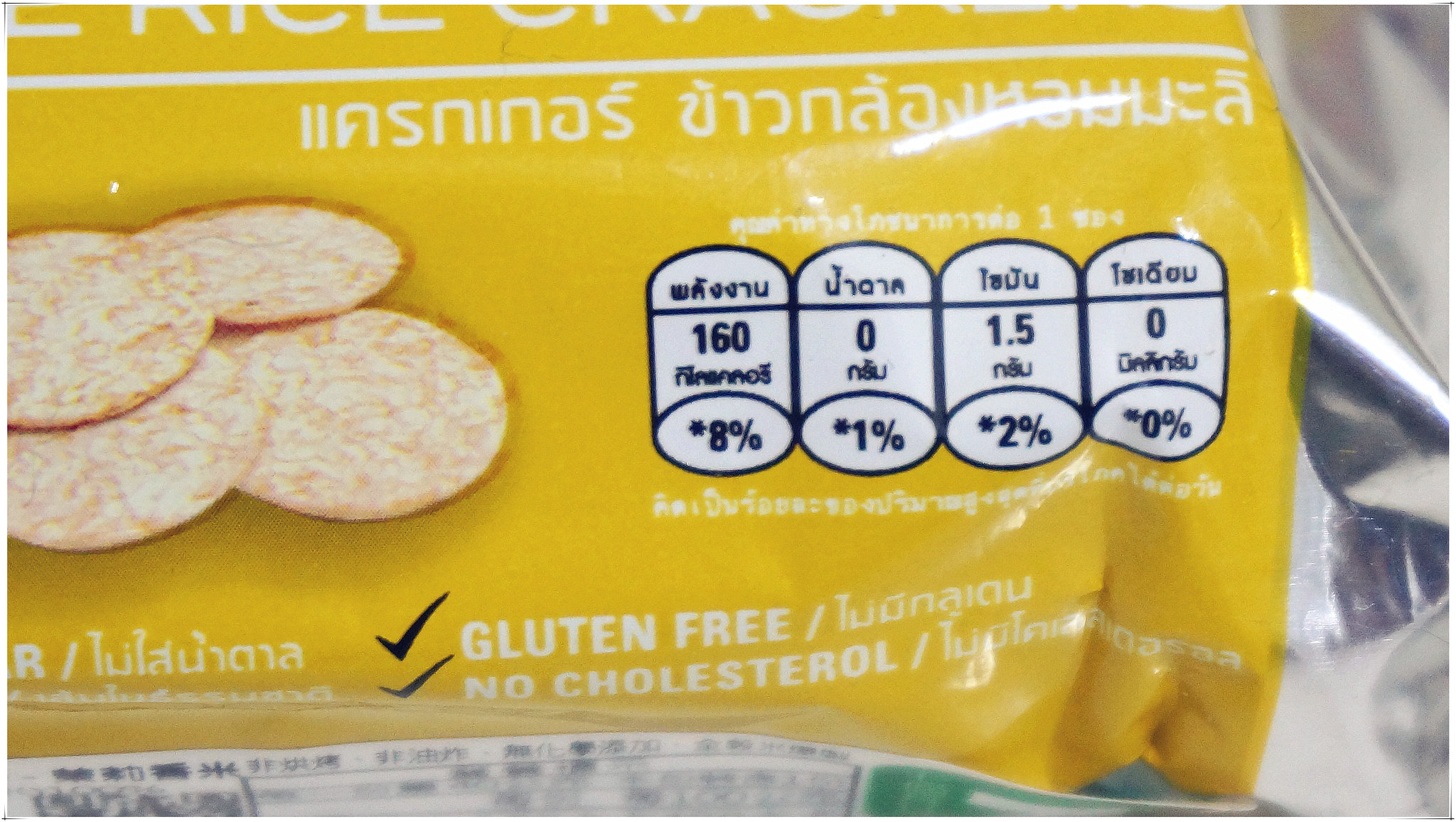This close-up image showcases a package of rice crackers. The package features a medium yellow tone and displays only a portion of the overall package. Specifically, it shows the bottom section, highlighting a photograph of four round rice crackers on the far left. These crackers are flat, thin, and have a light brown to white coloration, toasted around the edges, resembling wafer cookies. The packaging includes both foreign text and some English phrases, prominently stating "gluten-free" and "no cholesterol." White lettering and additional nutritional labels in the foreign language are also visible on the package. The image also depicts a section of a white napkin or place setting, along with what appears to be a silver spoon.